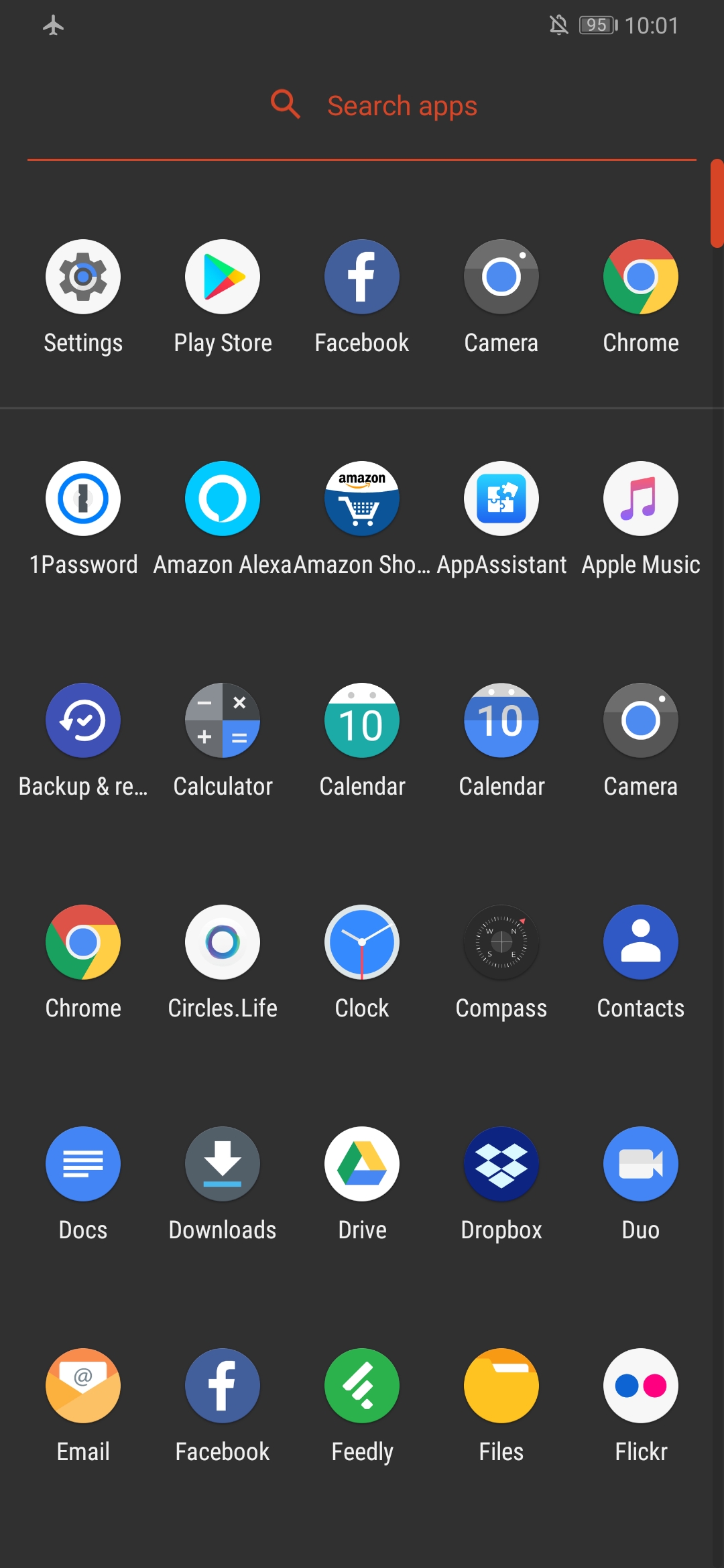The image depicts a screenshot of a smartphone's home screen, featuring a black background. At the top left corner, there is a small airplane icon indicating that the phone is in airplane mode. On the top right, a crossed-out bell icon signifies that the phone is in silent mode, and next to it, a battery symbol displays a charge level of 95%, indicating it’s nearly full. Further to the right, the time is shown as 10:01, without specifying AM or PM.

Beneath these indicators lies a red search bar with a magnifying glass icon, prompting the user to "search apps," along with a red underline. Below the search bar, there are six rows filled with five app icons each, totaling 30 icons. The apps are varied, encompassing common applications typically found on a main screen such as Settings, Google Play Store, Facebook, Google Chrome, Camera, Calculator, Calendar, Clock, Compass, Google Drive, and Flickr. All available spaces within these rows are occupied, with no blank spots visible.